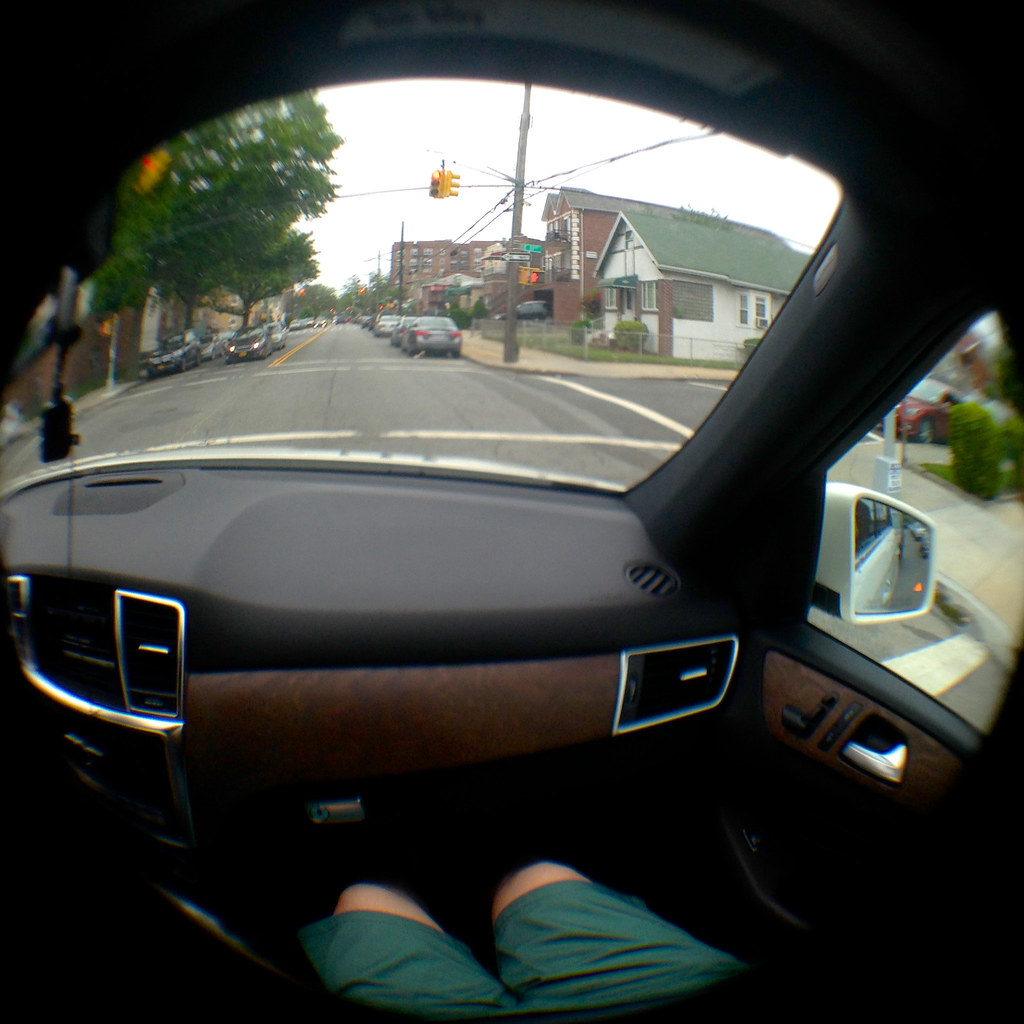In this daytime photograph, taken from the perspective of a passenger seated inside a vehicle, we observe the scene through a combination of black and brown wooden car interior. The lower part of someone's legs, clad in green shorts and appearing to be Caucasian, is visible from the hip to the knee, seated next to an air conditioning vent and a silver handle. Although the image is somewhat blurry and grainy, the exterior view through the car window reveals a street lined with parked cars on both sides. To the upper right, an old house sits at a corner, adjacent to a sidewalk. Beyond this, three- to five-story apartment buildings extend along the right side of the street. On the left side, green trees contrast with the oncoming traffic, contributing to the urban landscape depicted in the photograph.